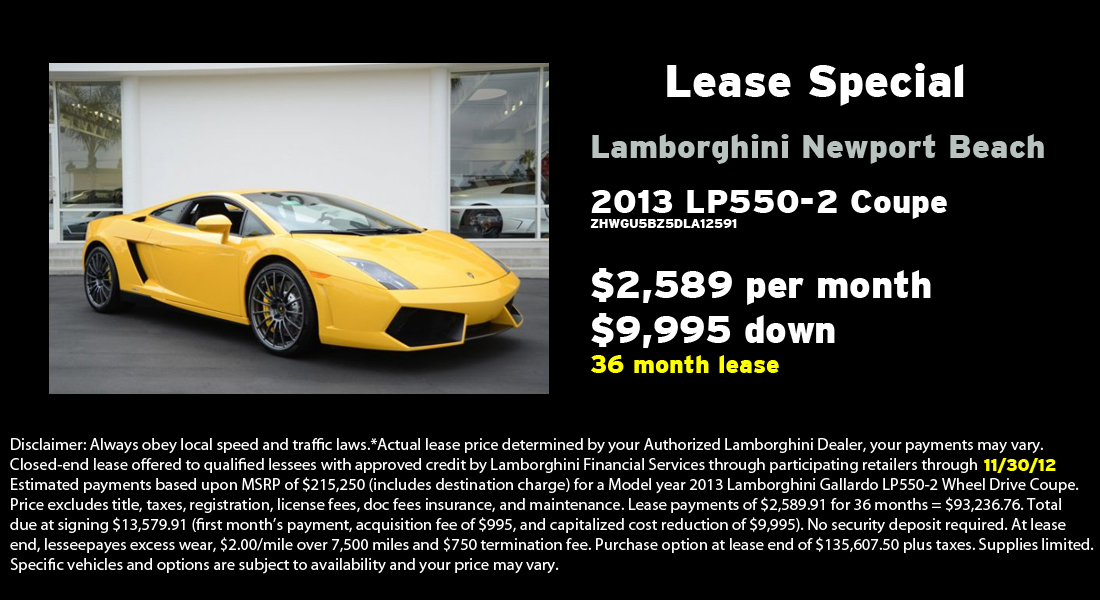An advertisement for leasing a Lamborghini at Newport Beach features a striking image of a sleek, yellow 2013 LP550-2 Coupe. The Lamborghini, characterized by its darker yellow color, big black wheels, narrow top, and sleek forward design, is prominently displayed on a clean asphalt surface in front of a white building with windows. Through these windows, you can observe additional white cars. The backdrop and car details present an appealing visual against a solid black upper left corner.

On the right side of the image, bold white text announces "Lease Special" with "Lamborghini Newport Beach" in gray letters below. Further details include the car's model number ZWHGU58Z5DLA12591. Pricing information follows: $2,589 per month with $9,995 down and a 36-month lease emphasized in yellow letters. A detailed disclaimer paragraph at the bottom, in smaller font, outlines terms and conditions, the vehicle's MSRP including destination at $215,220, and notes limited availability and conditions based on the model year and specific vehicle options. Payments vary and the offer is valid through 11/30/12. The right side text contrasts sharply against the dark background, drawing attention to the leasing details.